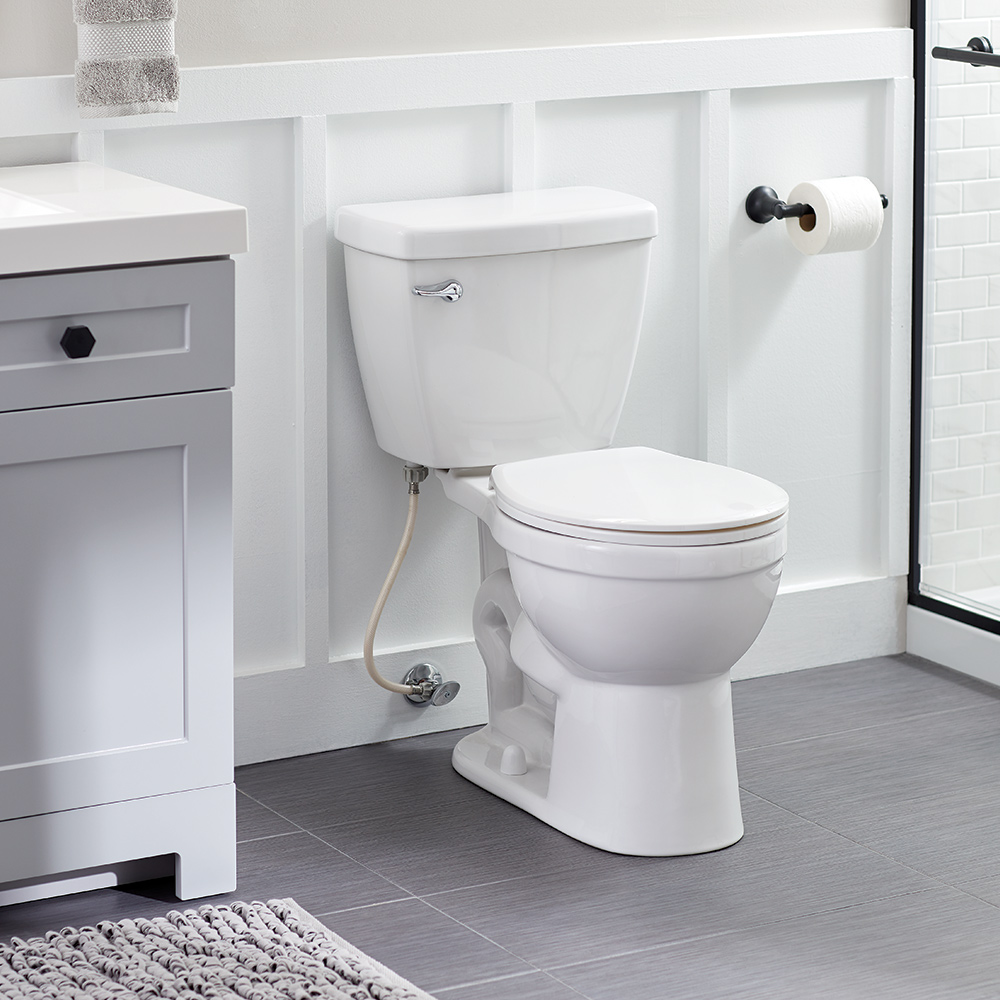The image captures a detailed view of a bathroom. Centered prominently is a white toilet, located to the left of a black toilet paper roll holder. Adjacent to the holder on the right is an open glass door leading into a brick-lined shower stall. On the left side of the toilet, there is a sink with a marble countertop, flanked by gray drawers and cabinet doors with black handles. At the top left corner, a light gray towel hangs, partially visible. The wall is predominantly white with wooden accents, with a base made of wood. In front of the sink and to the left of the toilet lies a gray shag carpet, complemented by a light gray rug and gray towels on the floor. The subtle interplay of gray and white tones creates a cohesive and elegant bathroom aesthetic.